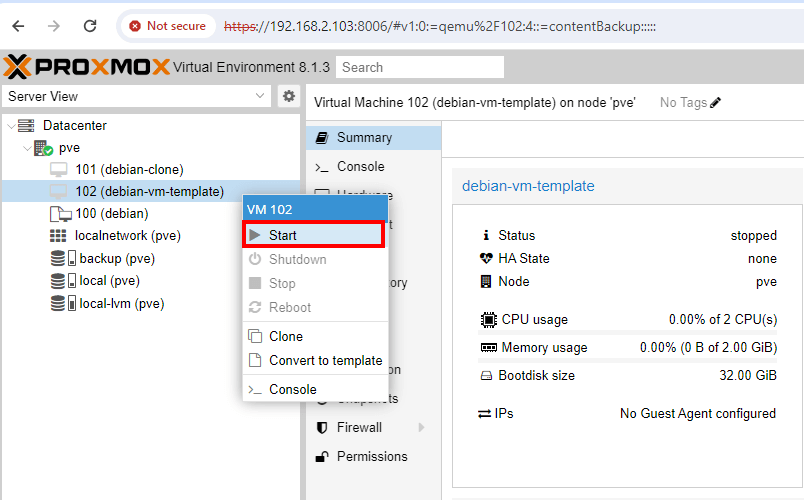This image is a large screenshot taken in portrait mode from a laptop. The visual elements are detailed as follows:

- **Top Bar**: 
  - **Upper Left Corner**: There is a back arrow along with a reload icon.
  - **Address Bar**: The URL shown is "192.168.2.103:8006" with a notification indicating "Not Secure."

- **Logo and Title**:
  - Just beneath the top bar, the background is dark gray.
  - **Logo**: Features an orange "X" behind a black "X."
  - **Title Text**: "ProXmoX" where "Pro" and "mo" are in dark black, and both "X"s are in orange.
  - **Version**: Reads "Virtual Environment 6.1-3."

- **Search Bar**:
  - Directly underneath the title, there is a search field.

- **Left Column**:
  - Multiple system categories are listed, including "Server View," "Data Center," and "PVE."
  - Network-related entries: "101," "102," "100," as well as "Local Network" and "Backward Local."
  
- **Pop-up Message**: 
  - Located between the left and right columns.
  - **Header**: Light blue color with the title "VM 102."
  - The first row in this pop-up is highlighted and surrounded by a thick red box displaying the text "Start."
  - Below the first row, options include "Shutdown," "Stop," "Reboot," "Clone," "Convert to Template," and "Console."

- **Right Column**:
  - The content pertains to "Virtual Machine 102."
  - Displays a summary labeled "DEBIAN VM Template."

This comprehensive description captures all the essential visual elements and textual information from the screenshot, presented in a neatly structured format.